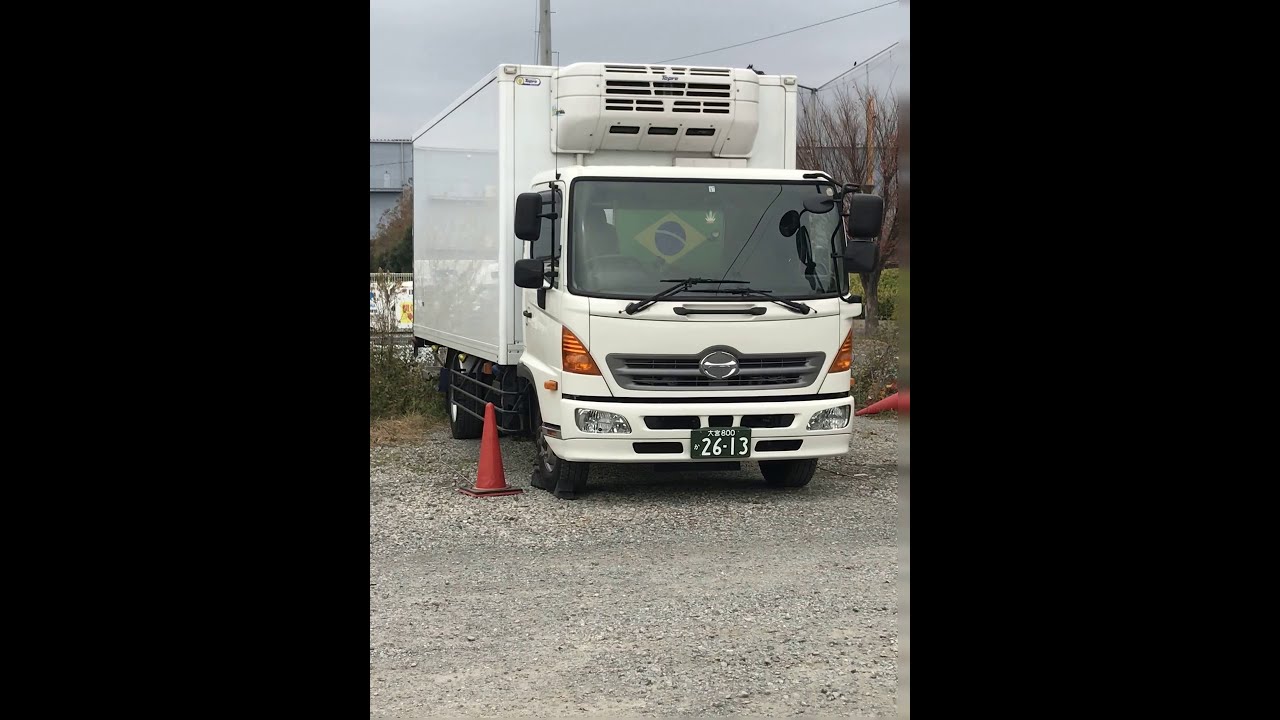A detailed full-color photograph captures a white truck, parked outdoors during the daytime on a gravel drive area. Thick black borders frame the image horizontally on the left and right sides. The truck, which appears large and might be built for transporting refrigerated goods, has a flat front tire on the passenger side. This is evidenced by the red traffic cone positioned next to the left front wheel and another similar cone lying tipped over on its right side.

A green license plate with Asian writing bearing the number 26-13 adorns the front bumper, indicating the truck's foreign, likely Asian, origin. Through the windshield, a Brazilian flag with a yellow diamond and blue circle stands out prominently, adding a splash of color and hinting at a connection to Brazil.

The background showcases a fence with bare tree branches and small bushes, while some grass, shrubbery, and power lines are visible, contributing to the rustic scene. The sky overhead is a dull gray, enhancing the overall somber yet intriguing atmosphere of the photograph.